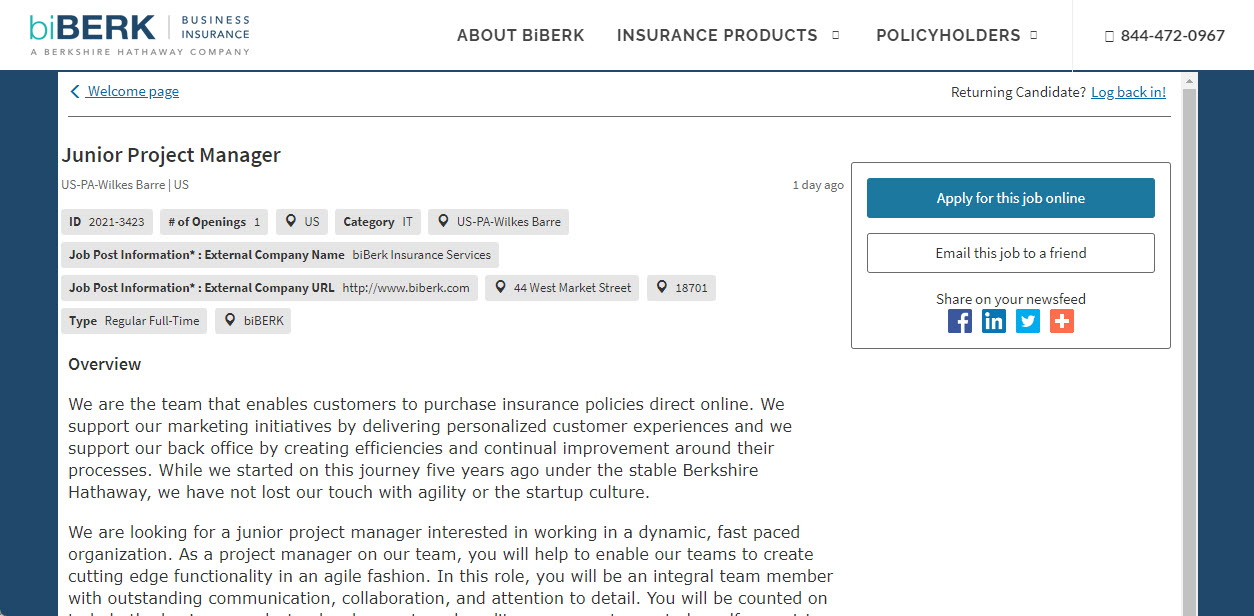This screenshot captures the homepage of the "By Burke" website, a subsidiary of Berkshire Hathaway, specializing in business insurance services. The top left corner features the "By Burke" logo, characterized by a distinctive lowercase 'b' and 'i' alongside an uppercase 'B-E-R-K'. The header includes navigation options such as "About By Burke", "Insurance Products", and "Policy Holders", clearly indicating the site's purpose of assisting users in managing or acquiring business insurance policies. 

A prominent contact number, 844-472-0967, is displayed at the top for customer support. As you scroll down, the site welcomes visitors and highlights a job opening for a Junior Project Manager. The job description points out that this role involves supporting the marketing team in a dynamic, fast-paced environment. The position requires strong communication, collaboration, and attention to detail to help the team develop cutting-edge functionalities in an agile manner. The page provides options to apply for the job online or share the opportunity via email and social media platforms such as Facebook, Indeed, and Twitter.